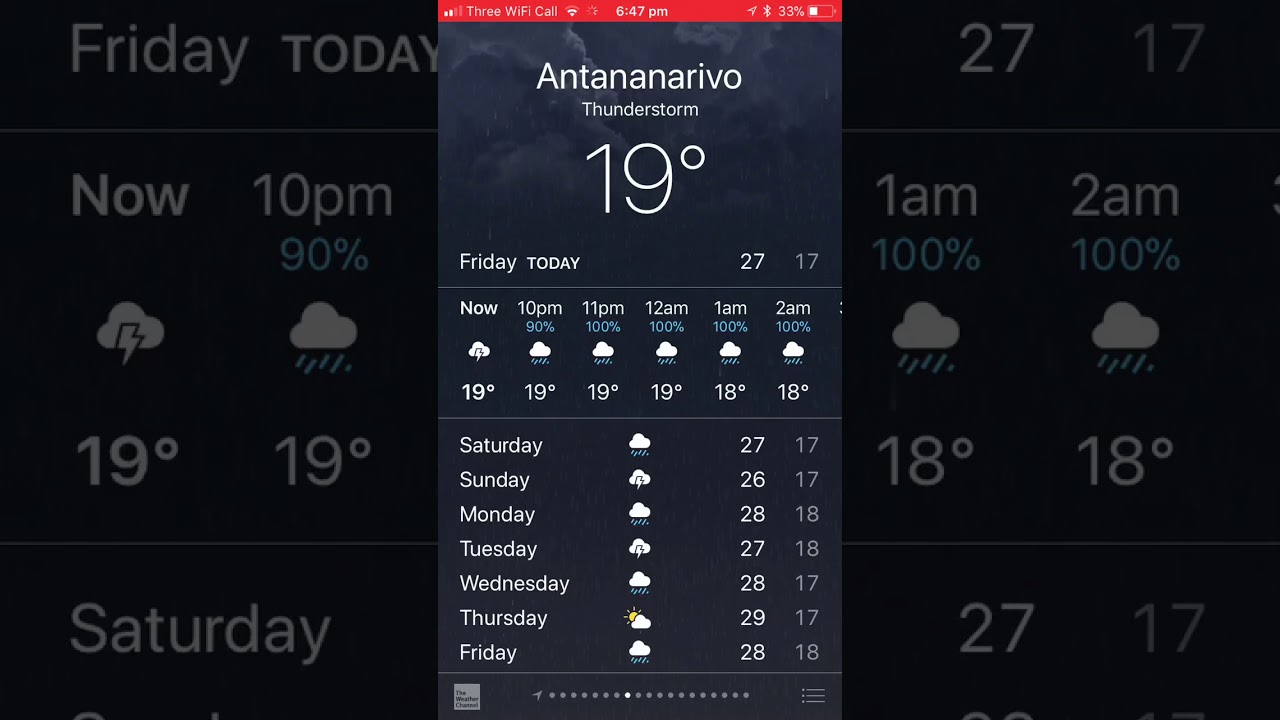In this detailed weather forecast image, the centerpiece resembles a smartphone screen displaying comprehensive weather information. At the very top of this central panel, a red bar frames icons for Wi-Fi, time (6:47 p.m.), and battery life (33%). The main weather details indicate an antenna icon, suggesting a thunderstorm with a temperature of 19 degrees. The forecast covers the present time (9 p.m.) through 2 a.m., showing a chance of precipitation at 100% for the initial hours and 90% for 10 p.m.

Beneath this immediate forecast, weekly weather predictions from Saturday through Friday are presented. The temperatures for these days are listed sequentially as 27, 26, 28, 27, 28, 29, and then 28 degrees, accompanied by weather icons indicating cloudiness, rain, and other conditions.

Flanking this central forecast screen, darker background panels provide additional weather details. To the left, a larger, zoomed-in view of the central forecast highlights minute details such as specific times of the day, temperature readings, and precipitation percentages under the heading "Friday Today."